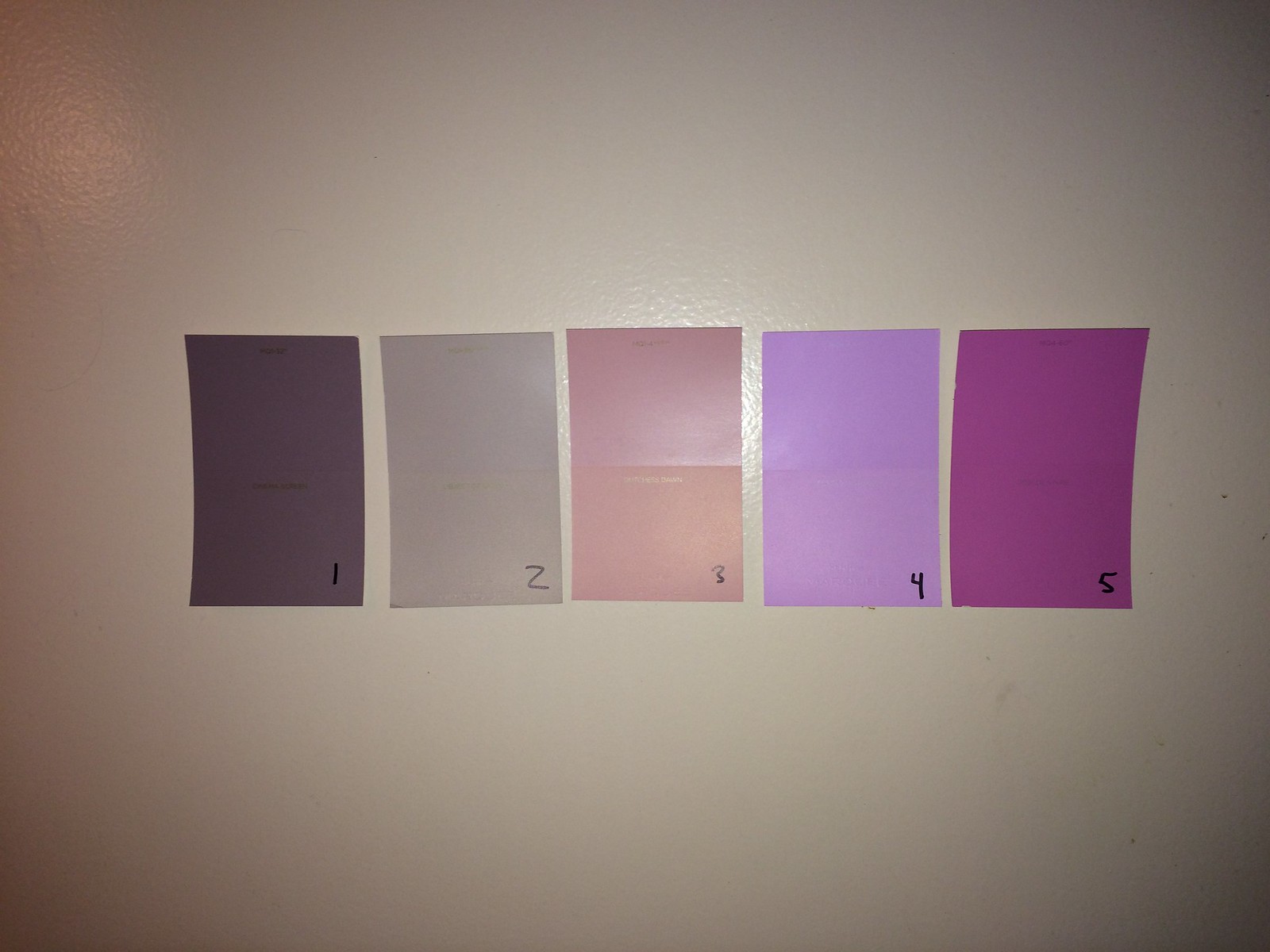The photograph features a solid white wall with a grainy, textured surface that reflects light, causing the center to appear lighter and the edges to look darker. Five paint swatches are aligned in the center of the image, each slightly curved outward as though they are not completely adhered to the wall. The swatches are numbered in black handwriting at the bottom right corners. 

The arrangement begins with a dark purple swatch marked with the number one. Next to it is a lighter, grayish purple swatch labeled with the number two. The third swatch in the sequence is pink and marked with a three. The fourth swatch is a vivid neon lilac purple with a four written on it. Finally, the fifth swatch is a rich purple color, designated with the number five. Despite some scuffs and imperfections on the wall, the array of colorful swatches create a visually intriguing juxtaposition against the reflective white background.